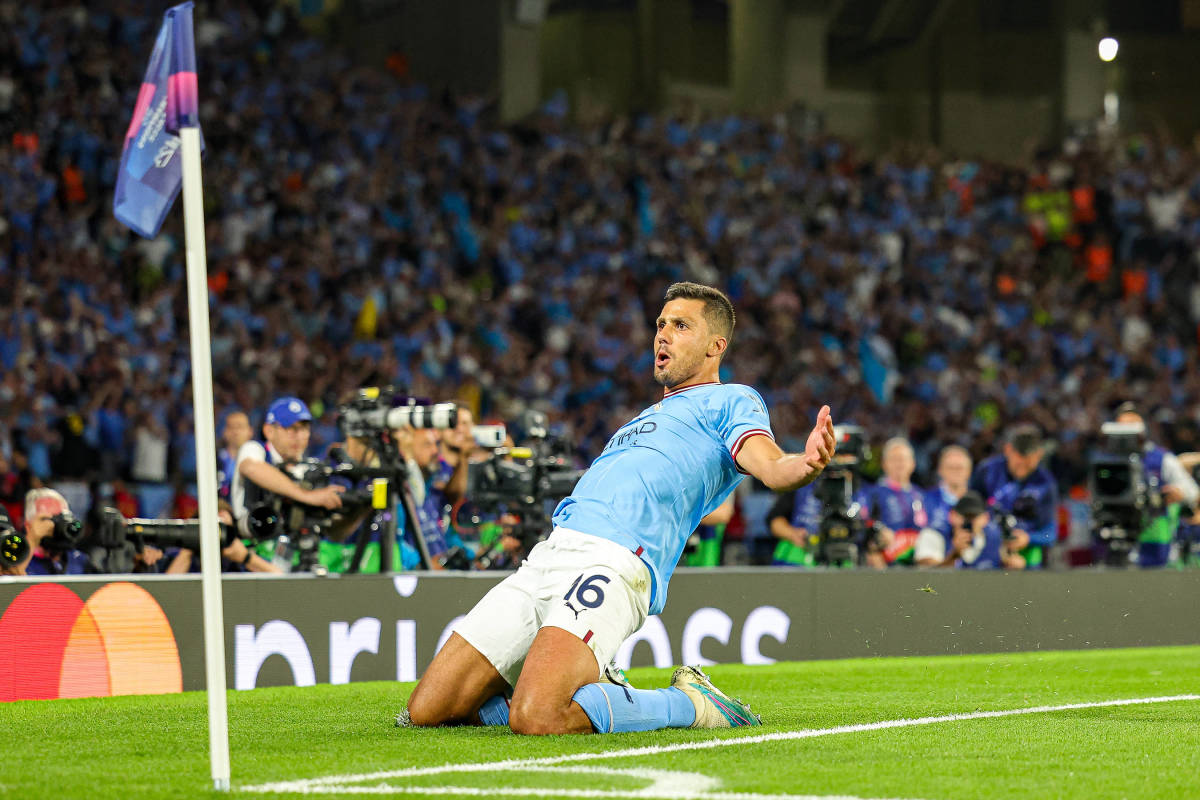In this image, we see a Manchester City soccer player celebrating on the field. He is wearing the signature Manchester City light blue jersey with red marks on the neck and sleeves. His jersey prominently displays the number 16. The player is in a joyful pose, sliding on his knees across the grass, suggesting that he was celebrating a significant moment, possibly a goal, even though his facial expression hints at uncertainty about the outcome.

He is also donned in white shorts and blue hose, with blue and white boots completing his athletic attire. The background reveals a vibrant scene with a large crowd of spectators, estimated to be around 10,000 people, filling the stands. Several high-quality cameras can be seen positioned around the field, capturing every moment for what could be high-paying action shots for media outlets.

In the corner of the field, we notice the pole and flag, along with visible markings on the ground. The combination of the player's emotional celebration and the bustling stadium atmosphere encapsulates the intensity and excitement typical of a high-stakes soccer match.